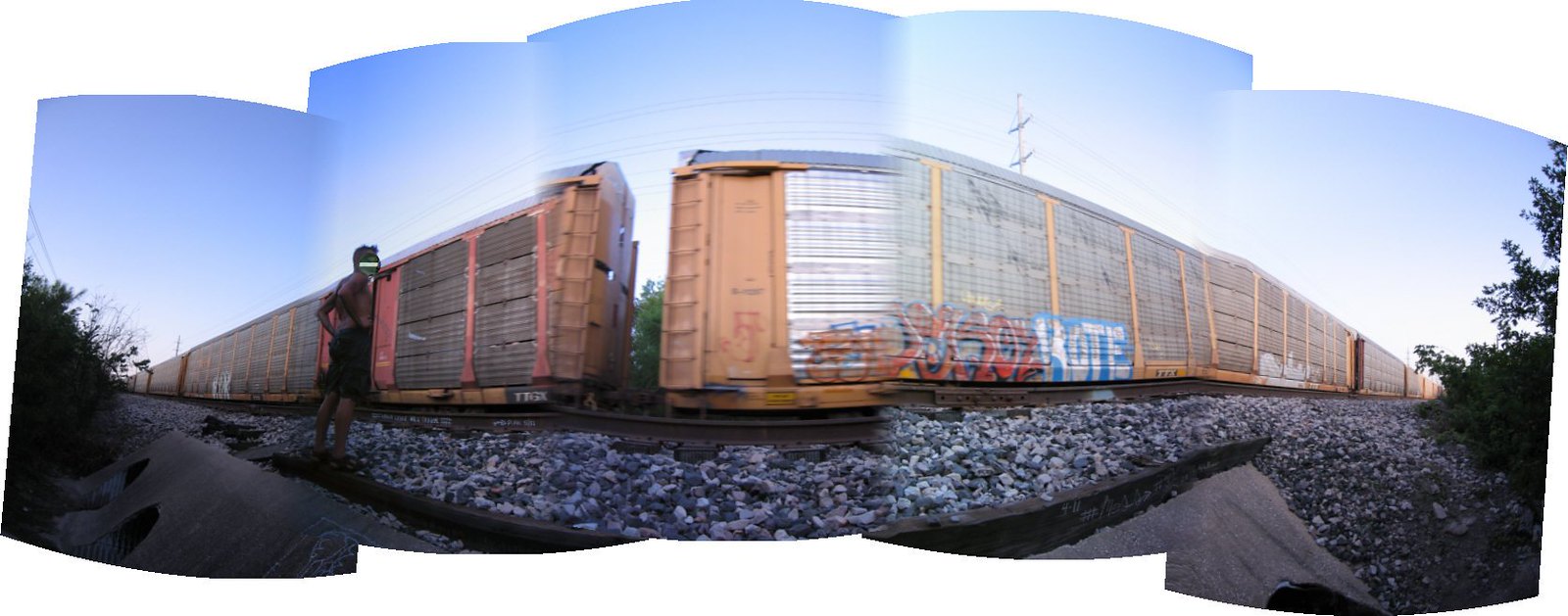The image depicts a slightly distorted panoramic view of a potentially abandoned, dingy cargo train covered in graffiti, including a prominent 'VOTE' tag in white lettering on a blue background. The train, mainly beige with hints of red, sits on tracks surrounded by gravel and stones. The stitching of the panoramic photo creates a warped perspective, with the train appearing largest at the center and tapering off towards the edges. The scene is bright with a clear blue sky, indicating daytime. To the left of the frame, a shirtless person in dark shorts stands, looking towards the train. Additional details include trees on either side and a distant telephone pole, completing the industrial and slightly desolate atmosphere.